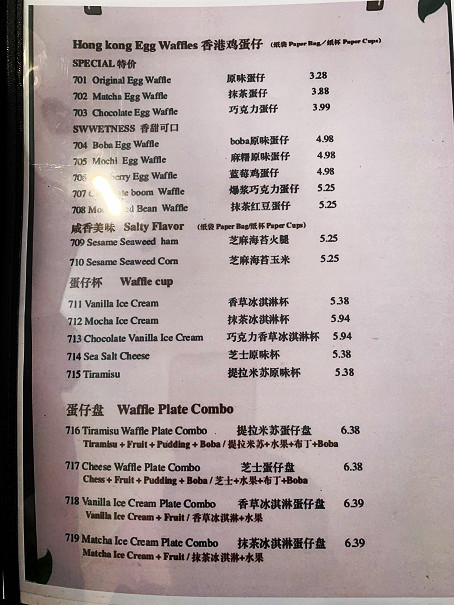The menu presented is printed on white paper featuring black text. It is organized into several categories, each showcasing a variety of Hong Kong egg waffles. The menu includes detailed entries for different types of waffles, each with the dish name in Chinese and the corresponding price listed nearby.

Starting with the **Special Waffles** category, the options include:
- Original Egg Waffles
- Matcha Egg Waffles
- Chocolate Egg Waffles

Following this section, the **Sweet Waffles** category offers:
- Boba Egg Waffles
- Mochi Egg Waffles
- Strawberry Egg Waffles
- Chocolate Boom Waffles
- Bean Waffles

Next, the **Salty Flavor Waffles** category features:
- Sesame Seaweed Ham Waffles
- Sesame Seaweed Corn Waffles

In the **Waffle Cups** category, the menu lists:
- Vanilla Ice Cream
- Mocha Ice Cream
- Chocolate Vanilla Ice Cream
- Sea Salt Cheese
- Tiramisu

Finally, the **Waffle Plate Combos** category includes:
- Tiramisu Waffle Plate Combo
- Cheese Waffle Plate Combo
- Vanilla Ice Cream Plate Combo
- Matcha Ice Cream Plate Combo

Each dish name is also provided in Chinese characters alongside the English names, accompanied by their prices, ensuring ease of understanding for all customers.